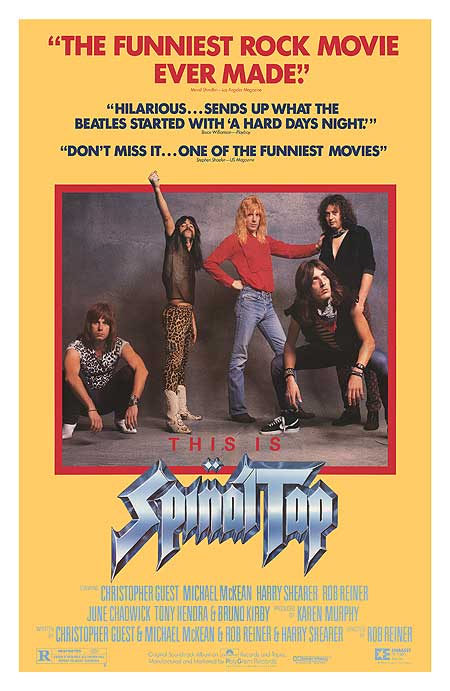This promotional poster for the film "This is Spinal Tap" features a predominantly yellow background that transitions from darker at the top to lighter at the bottom. At the top, bold red text proclaims it as "The Funniest Rock Movie Ever Made," while black text below emphasizes its comedic appeal with quotes like "Hilarious. Sends up what The Beatles started with A Hard Day's Night" and "Don't miss it. One of the funniest movies." A central, red-bordered image showcases the five flamboyantly dressed members of the fictional rock band Spinal Tap. The band members, all sporting long hair, strike various poses; one in a black outfit crouched, another standing in black, a third in a red shirt with blue jeans and blonde hair, a fourth in leopard print with a sheer top and raised fist, and the last in a white and black patterned top with feathered hair, also crouched. The band's name, "Spinal Tap," appears in embossed metal-style print below the image, accompanied by the names of the actors and the director in lighter blue text. The film is rated R, and the overall design evokes a rock-n-roll vibe suited to the film’s mockumentary style.